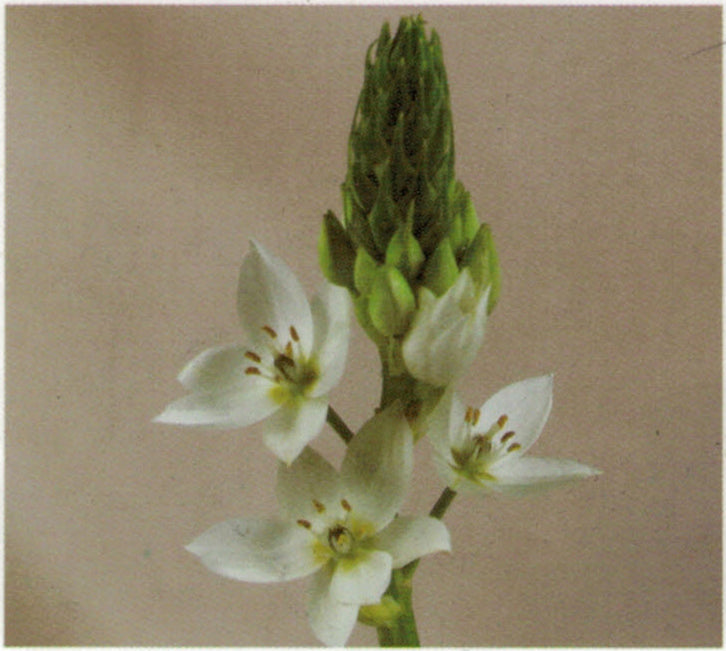This photograph showcases a cluster of small white Star of Bethlehem flowers on a green stem, set against a light tan or beige background. The image, enclosed within a thin white border, is somewhat blurry with noticeable visual noise. The flowers feature pointy petals, typically numbering six, with three fully bloomed and one beginning to open. Yellow filaments and pollen are visible at the center of each blossomed flower. Above these, the stem bears several unopened green buds resembling pine cones.